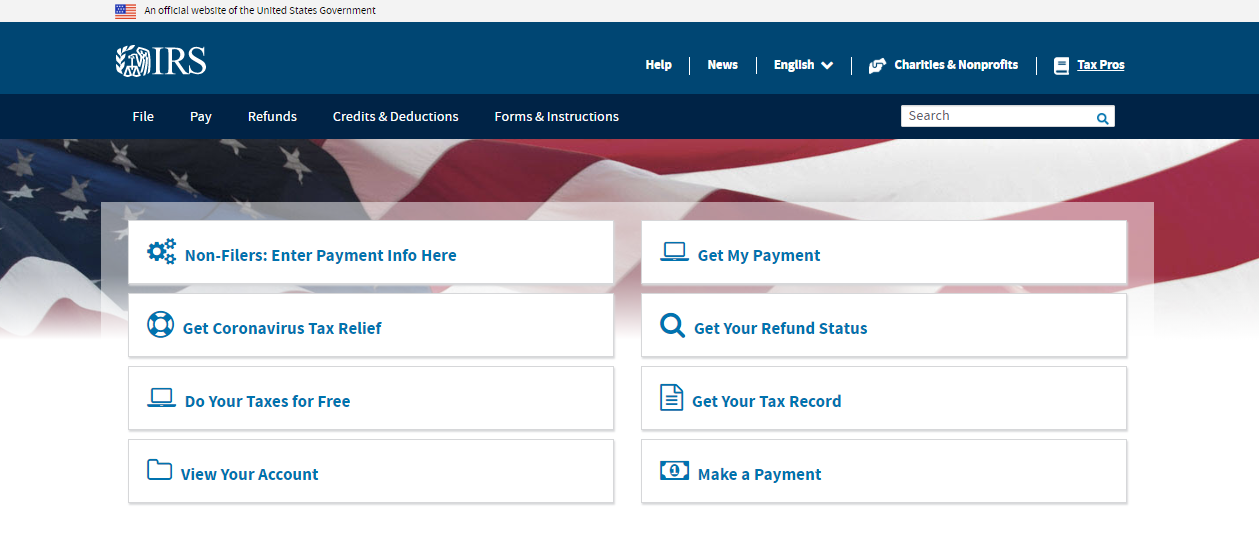A screenshot of the IRS website's homepage is displayed, capturing a significant portion of the interface. The layout prominently features typical IRS-related services such as "Tax Relief," "Do Your Taxes for Free," "View Accounts," "Get My Payment," "Refund Status," "Get Your Tax Record," and "Make a Payment." The design maintains a conventional and subdued aesthetic, predominantly utilizing a patriotic color scheme of red, white, and blue. A modest blue banner at the top houses the IRS logo in white text. The site appears straightforward and utilitarian, designed to facilitate various tax-related tasks for users.